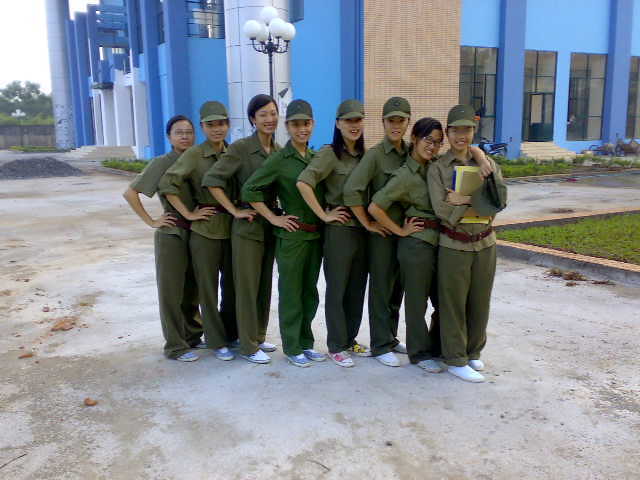The image features a line of eight smiling Asian women standing one behind the other, each with their right hand on their hip, and dressed in varying shades of green. They're wearing long green pants ranging from khaki to gray-green, with brown leather belts around their middles. Their tops include long-sleeved shirts that are either rolled up to the elbows or three-quarter length, also in green hues. They all have flat sneakers in different colors, including white, blue, and red, with one pair featuring a unique red and yellow floral design on opposite sides. Five of the women are wearing hats, and one woman in the front has her arms crossed, holding a yellow notebook. The scene is set in front of a modern, bright blue-painted building with darker blue columns and some exposed brown brick. The women stand on a concrete parking area, and there's a distinctive old-fashioned lamppost with five globes on wrought iron arms nearby. Overall, the bright and cheerful atmosphere, combined with the mixed uniforms and their happy expressions, suggests a casual workplace setting rather than a military environment.